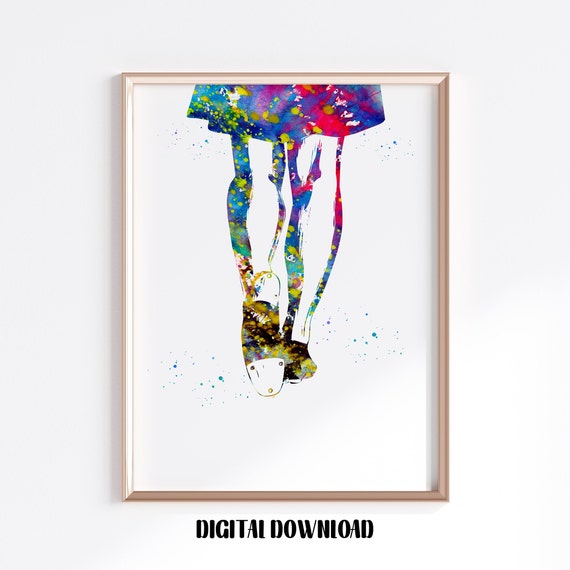The image displays a digital art piece designed to mimic watercolor, mounted on a white wall. The artwork is framed in a light pink frame that encases a vibrant, color-rich painting. The top part of the painting showcases a wider, abstract shape composed of blue, green, yellow, and red hues, from which multiple lines in various colors, including blue, green, and red, descend. These lines culminate in a pair of dangling legs, which appear to belong to a female figure, as evidenced by the glimpse of a skirt at the top. The feet are depicted in brown, yellow, and white tones, resembling a shoe-like form. Below the painting, the words "DIGITAL DOWNLOAD" are inscribed in black capital letters, bringing a modern touch to the overall presentation. The entire setup rests against a plain white background, emphasizing the vivid colors and the contemporary style of the piece.